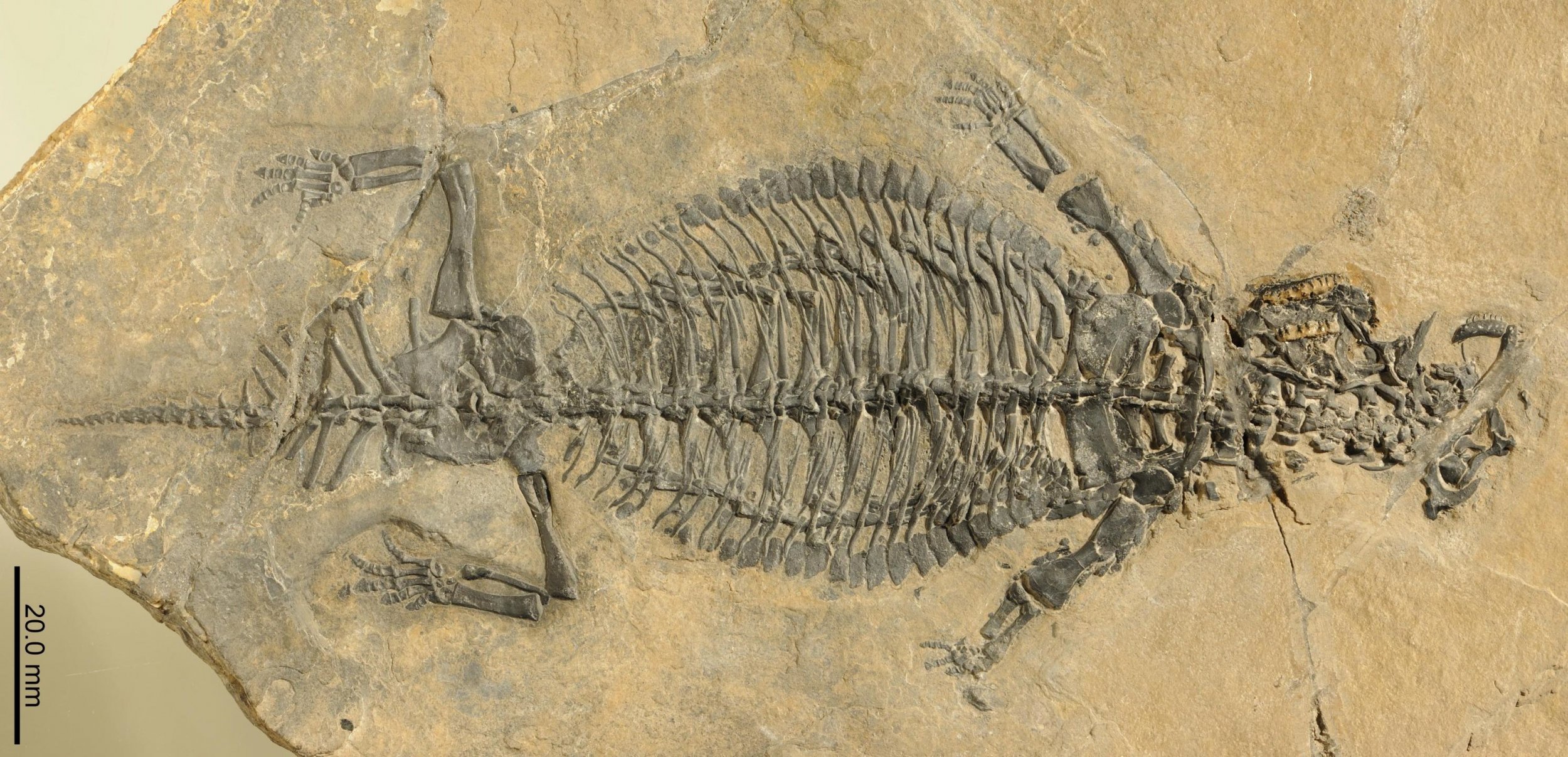The photograph showcases a fossilized skeleton embedded in a brownish-gray, speckled stone slab, which features noticeable cracks. The fossil, primarily dark gray to light gray, depicts a creature reminiscent of a lizard or crocodile. The skeleton's intricate details, including a large abdomen, two front legs, two back legs, and a wide tail, are clearly outlined. A scaling line in the bottom left corner indicates a measurement of 20.0 millimeters, suggesting the fossil's small size. The head of the creature is indistinct, making it challenging to identify the exact species. This image could easily belong in a museum display, offering a glimpse into the ancient past.